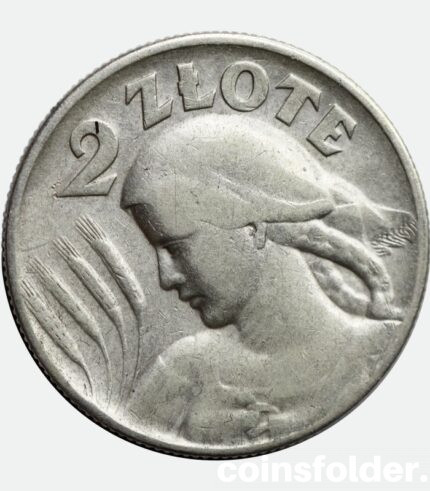The image depicts a round, silver coin set against a light gray background. The coin features the profile of a woman with braided hair and a headdress, looking towards four wheat heads on her left. Above her head is the number "2," and the letters "Z-L-O-T-E" encircle her profile, indicating its denomination as "Two Złote." The coin's edges are textured with a rough, diamond-like pattern. At the bottom right corner of the image, the phrase "coins folder." is displayed, suggesting it might be an advertisement or categorization for a collection. The coin appears well-worn, which adds to its aged appearance.